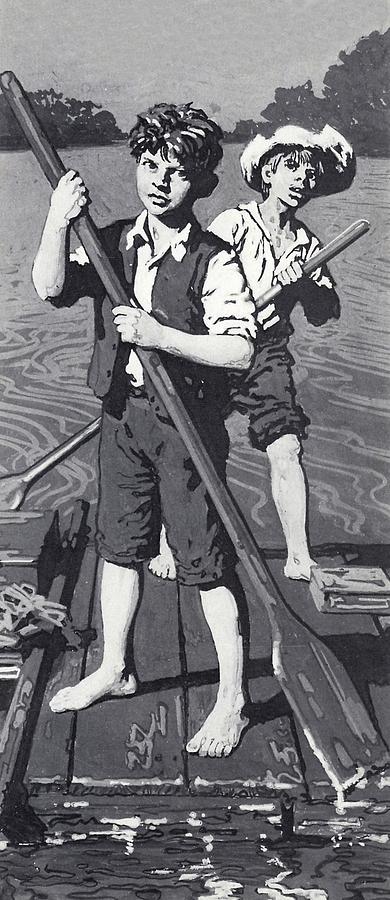This detailed black and white illustration appears to be a traditional painting that might depict characters from Mark Twain's classic novels, Huckleberry Finn and Tom Sawyer. In the drawing, two boys are paddling a somewhat complicated wooden raft down a river, presumably the Mississippi River. The scene, likely set in the early 1900s, captures the essence of rural adventure. The larger boy at the front, identified as Tom Sawyer, is wearing a dark vest over a white shirt, with dark pants that are rolled up. He gazes directly toward us with his oar in hand, showcasing his messy hair. Behind him stands Huck Finn, a blonde-haired boy sporting a white shirt and a straw hat, also with dark pants rolled up just above the knee. The background reveals the river flanked by trees on either side, suggesting a serene but adventurous setting. There is also a book visible on the raft, adding to the narrative that these boys might be on one of their many escapades. No additional information, artist signature, or text is present in the illustration to provide further context.